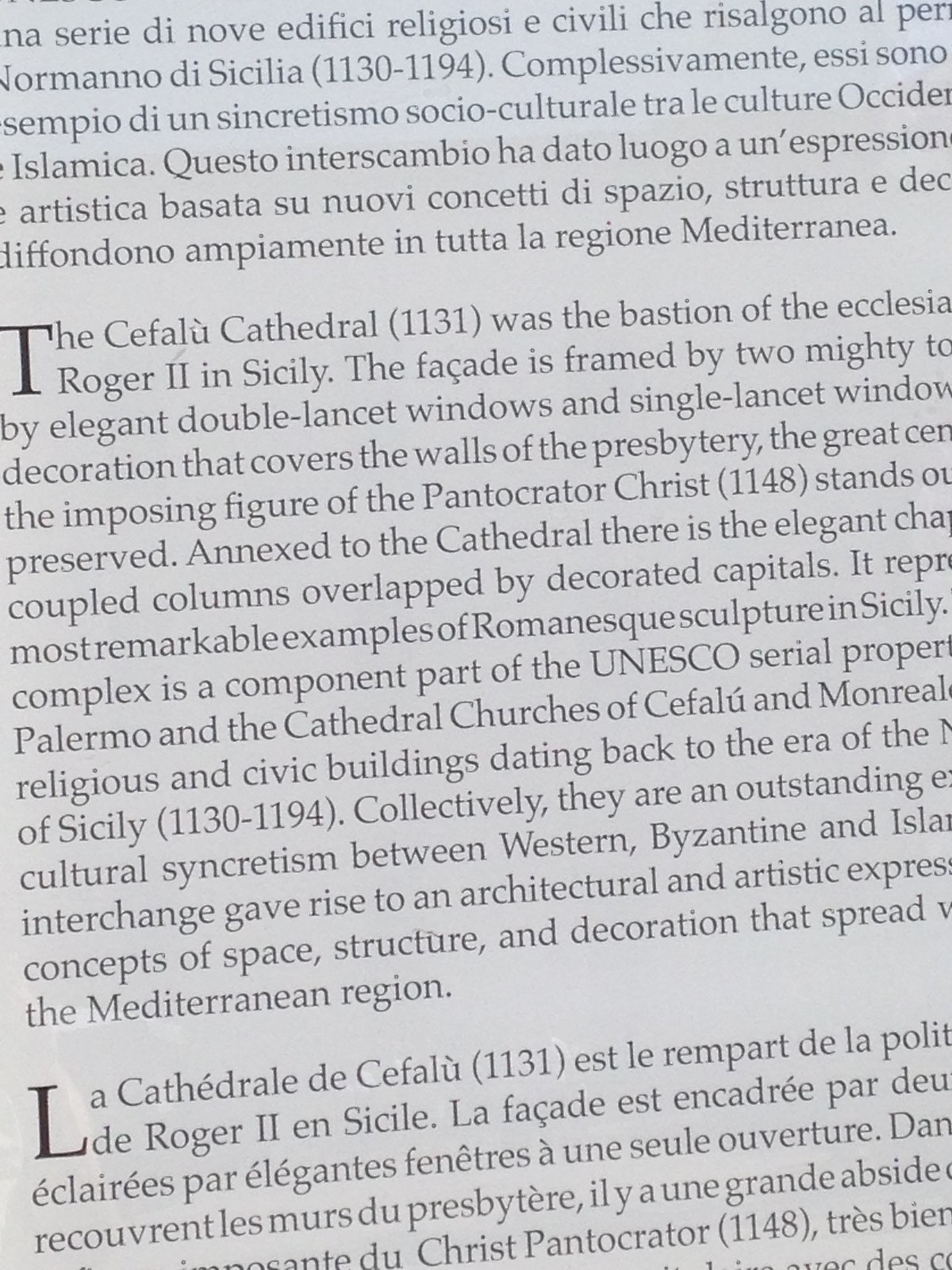The image displays a partially visible page, possibly an excerpt from a book or a religious text, most likely in Italian. The page, a shade of white to grey, features black text with the distinguishing attribute of each paragraph having a prominently larger and bold capitalized first letter, such as the "T" in the second paragraph and the "L" in the last. Only parts of the paragraphs are visible due to the page being cut off on the left, top, right, and bottom edges. The text includes words and phrases such as "cathedral," suggesting it describes architectural elements or historical topics, potentially about Sicily. Specifically mentioned within the fragmented text are descriptive elements like the Cefalù Cathedral, Roger II in Sicily, its façade, elegant double lancet windows, and the notable Pantocrator Christ from 1148. The contents combine cultural and architectural descriptions, highlighting the interconnectedness of socio-cultural expressions in historical contexts.